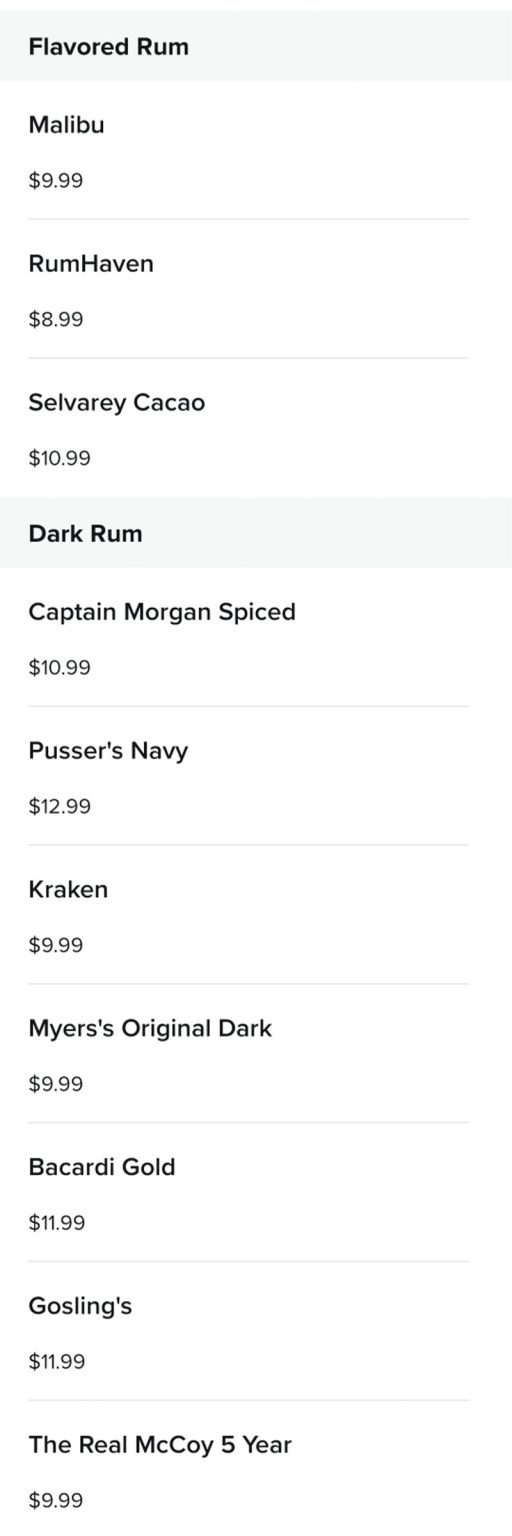The image features a primarily white background with two distinct light blue boxes at the top and in between, separating different categories of rum. In the first light blue box at the top, the text "Flavored Rum" is written in black print. Below this heading, the list of flavored rums and their prices interspersed with thin lines are as follows:

- Malibu for $9.99
- Rum Haven for $8.99
- Silbury Cacao for $10.99

Beneath these listings, there is another light blue box with the heading "Dark Rum" in black print. The dark rum selections and their prices, also separated by thin lines, include:

- Captain Morgan Spiced for $10.99
- Pusser's Navy for $12.99
- Kraken for $9.99
- Myers Original Dark for $9.99
- Bacardi Gold for $11.99
- Gosling's for $11.99
- The Real McCoy Five Year for $9.99

The overall image presents a clear categorization and pricing of various flavored and dark rums.